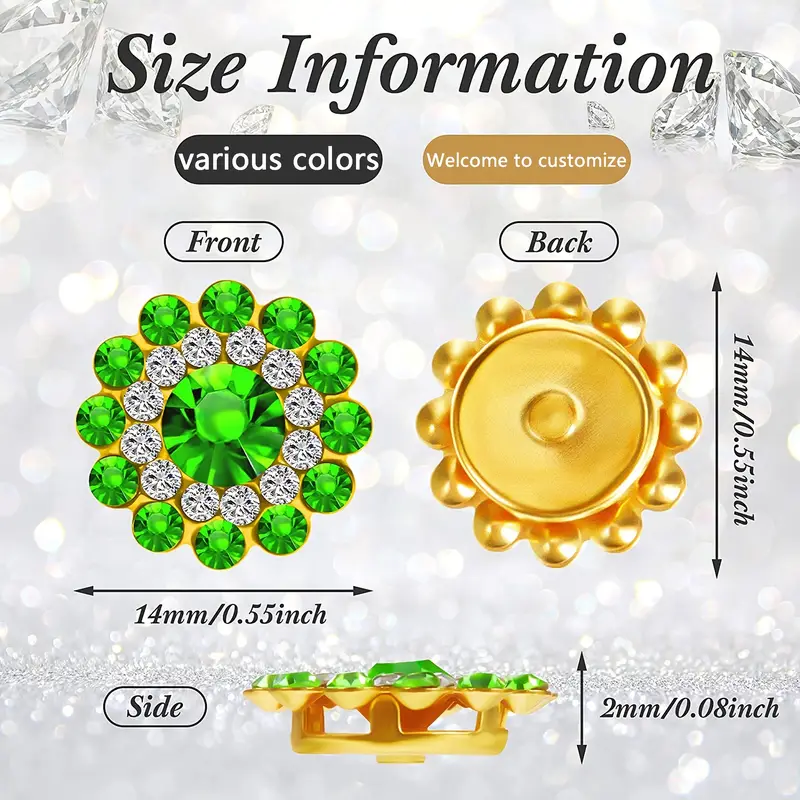This square image showcases an exquisite piece of jewelry. The back of the piece is crafted in gold and adorned with small circular details along the perimeter. The front features an intricate setting with a large, vibrant green gem at the center, surrounded by a series of dazzling white diamonds. Encircling the diamonds are additional smaller green gems, completing the luxurious design. 

The side view reveals the three-dimensional nature of the piece, which is elevated on small legs, offering a glimpse of the underlying structure that supports the arrangement of gemstones. 

Prominently displayed at the top of the image in bold black letters is the heading "Size Information." Below this, blocks of text indicate options for "Various colors" and "Welcome to customize," emphasizing the customizable nature of the jewelry. The image thoughtfully labels the front, back, and side views, and includes detailed dimensions of the piece to provide a comprehensive understanding of its size.